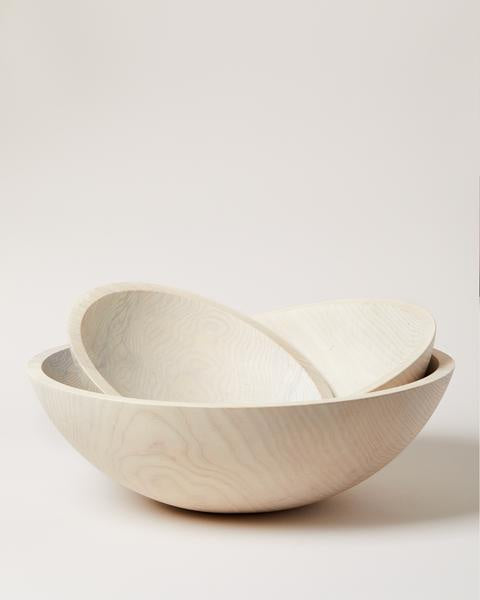The photograph showcases a vertically aligned rectangular image with a solid beige background, blending seamlessly with the surface, possibly achieved through studio lighting. The image features a large, light wooden bowl with slightly darker, tan-hued grain patterns, giving it a natural and premium look. Inside this large bowl are two smaller wooden bowls, each meticulously crafted from the same light wood with subtle, darker grain textures. The bowls are arranged at different angles within the larger one, creating a visually appealing composition. The simplicity of the background highlights the elegant texture and intricate grain of the wooden bowls, making them stand out as sturdy and beautifully designed pieces.